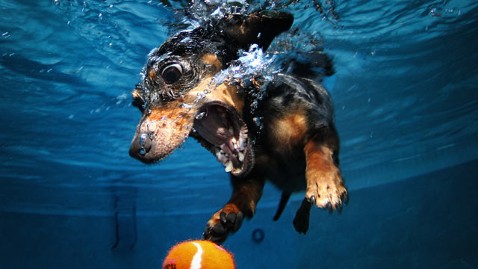This distinctive, horizontally aligned rectangular photograph captures a humorous and captivating underwater scene. It features a small dog, likely a dachshund, with a brown face and paws and a black body, mid-dive in a pool, attempting to retrieve an orange and white tennis ball. The dog's mouth is wide open as it eagerly tries to catch the ball, its bulging eyes reflecting its determination. Bubbles trail from its mouth, intensifying the comic effect. The top of the image showcases the water's surface, with slight backlighting creating beautiful blue swirls. As your eyes move downward, the image darkens, reflecting the deeper water. You can also see splashes indicating the dog's recent dive. The background reveals the pool's bluish-gray wall, featuring a vent and part of a ladder on the left side. The photograph beautifully captures the amusing and intense moment of the dog’s underwater chase.